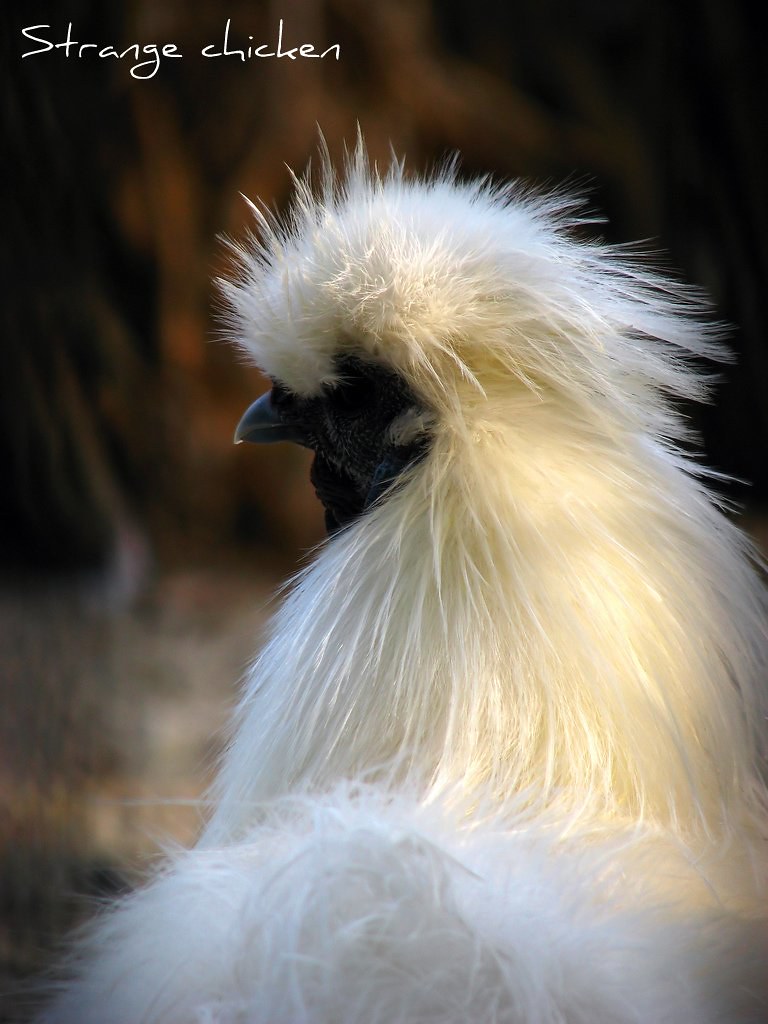The photograph in question is a close-up of a bird, prominently occupying the bottom right corner and extending upwards, making it the central focus of the image. The bird, likely a type of chicken, has distinct features including a black beak, a black face with black eyes, and what appears to be a black gobble. Its plumage is characterized by long, smooth, white feathers that puff out all over its body and head, giving it a fluffy, almost ethereal appearance. The bird is staring off to the left, creating a contemplative or curious expression. The background of the photograph is dark and hazy, adding a sense of mystery and making the bird's white plumage stand out even more. This blurry backdrop is a mixture of black and yellowish hues that may resemble hair or hay, contributing to the overall enigmatic feel of the photograph. At the top left corner of the image, the inscription "strange chicken" is written in italicized, white letters that resemble chicken scratch. This brief label adds a whimsical, yet ambiguous element to the image, encouraging viewers to question and interpret the nature of the bird they're observing.